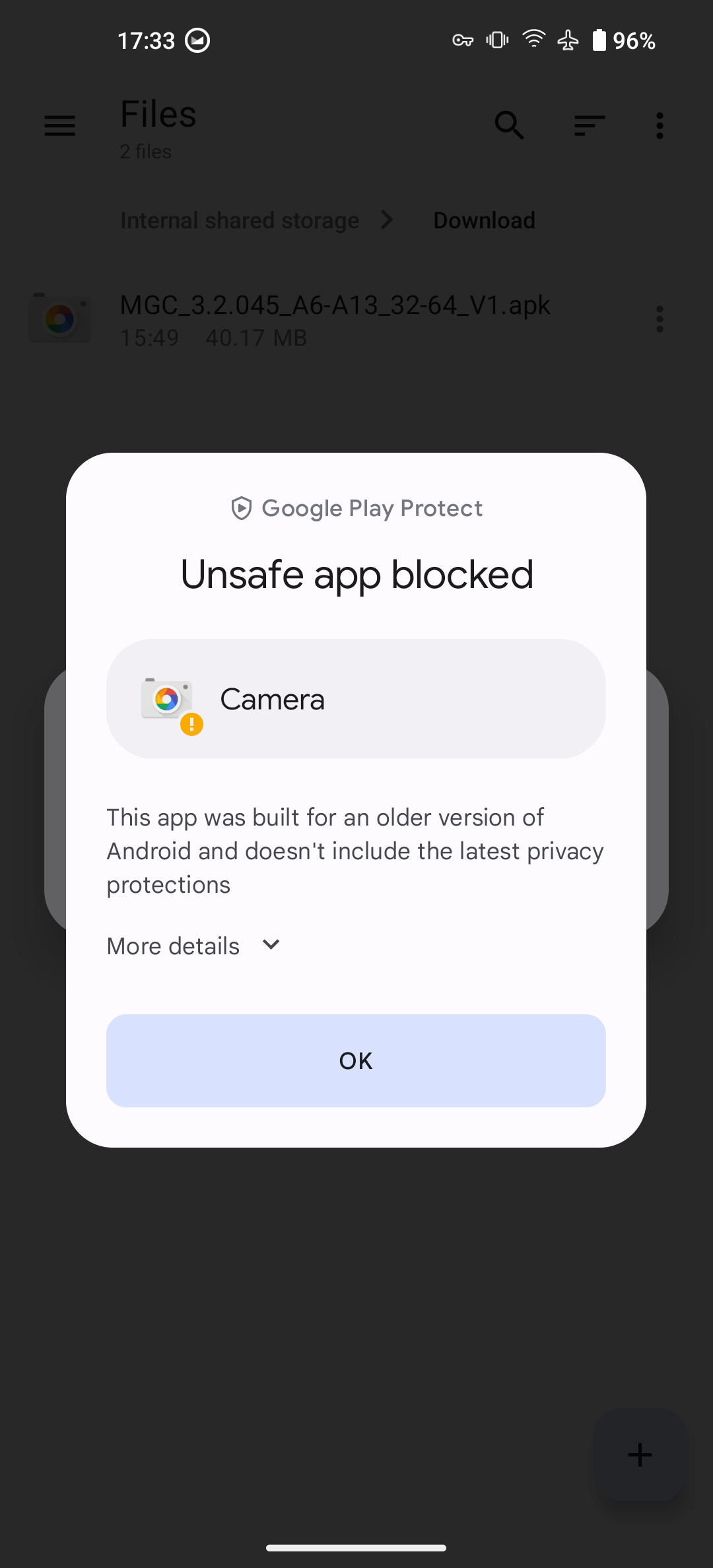The image displays a screenshot taken from a mobile device. The background is primarily grayed out, but faint black text is still visible. At the top, the text reads "FILES." Below that, the text displays "INTERNAL SHARED STORAGE," followed by an arrow pointing right to the word "DOWNLOAD." Further down, a string of alphanumeric characters is visible, reading "MGC3.2.045 A6-A13.332.64 V1.APK."

Underneath this string of characters, a small white pop-up window emerges. The pop-up message from Google Play Protect states, "Unsafe App Blocked." The message elaborates that the application in question, related to the camera, was built for an older version of Android and lacks the latest privacy protections. The pop-up concludes with an option to view "More details."